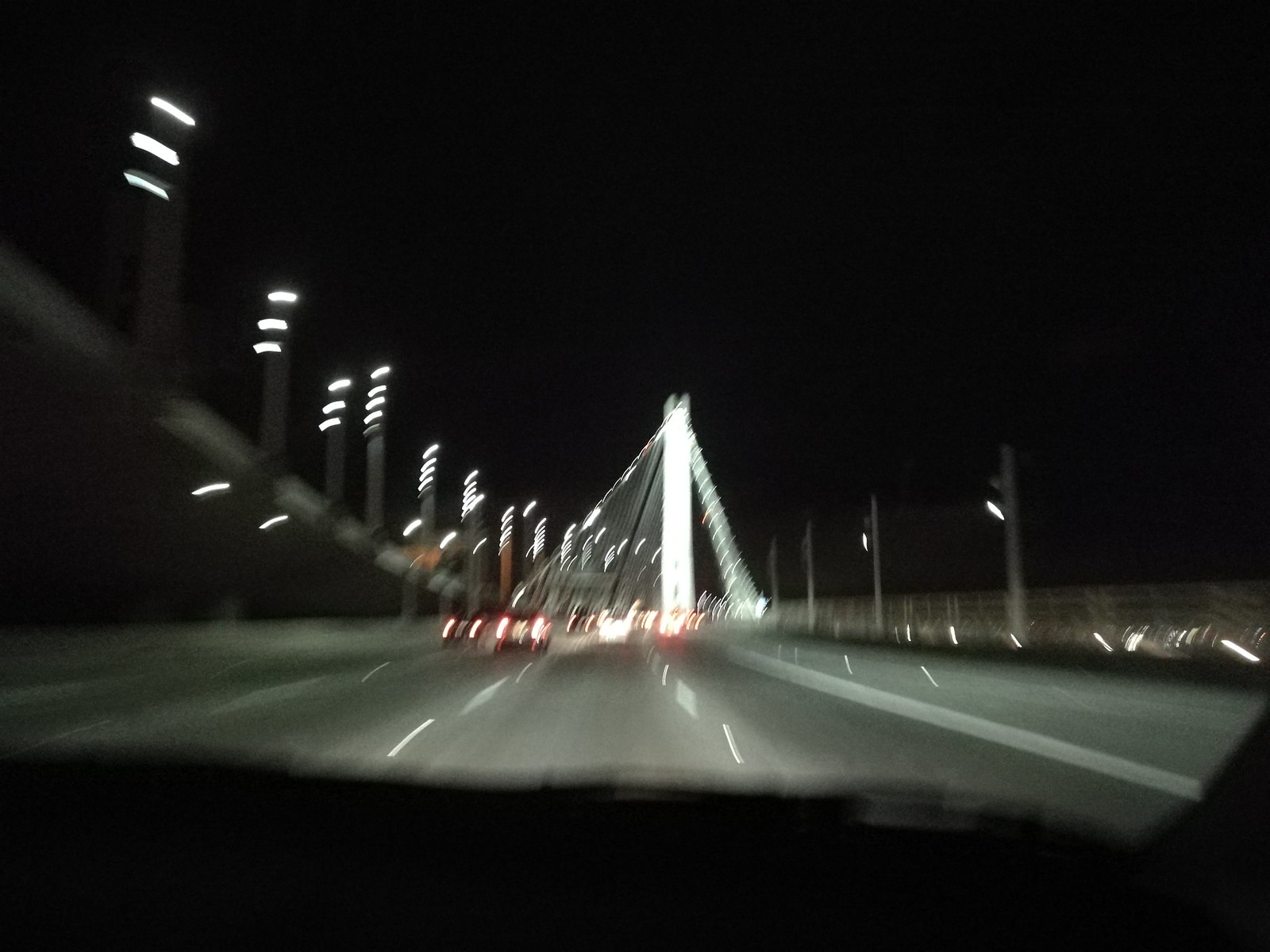This nighttime image, captured from the inside of a car, presents a driver's perspective on a multi-lane highway spanning a bridge. The sky is pitch black, void of stars or the moon. The scene is illuminated by numerous taillights of cars ahead, creating a trail of red light through the photo. The image is blurred, giving it a distorted and abstract quality, with the lights streaking into elongated shapes. Street lamps and road lights line the sides of the road, ensuring it is brightly lit. A towering bridge column can be seen with tension cables stretched downwards, and possibly metal fencing along the edges, confirming the bridge setting. Lane markings are visible, with a broken line on the left and a solid white line on the right, indicating no passing. The car appears to be positioned in the middle lane, navigating through the illuminated, albeit blurry, highway at night.